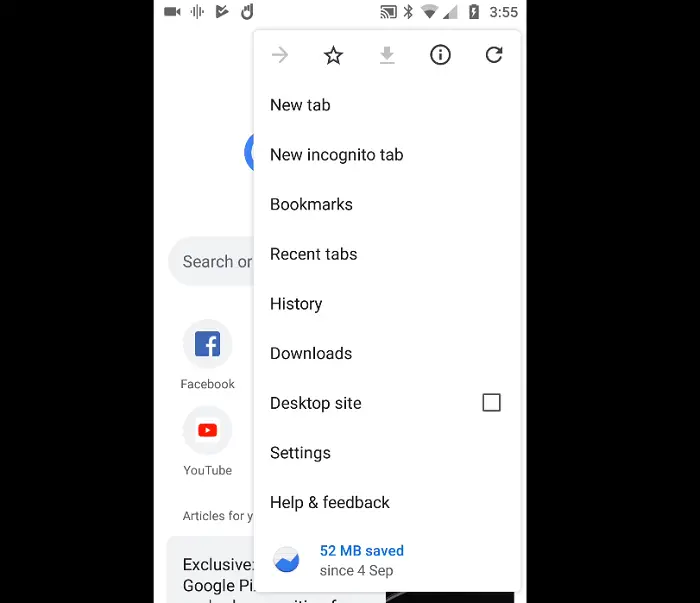The image showcases a cell phone screen superimposed on a black rectangle background, rendering the overall image nearly square with black borders flanking either side of the white cell phone screenshot. The phone's status bar at the top displays several icons including a movie camera, a sound icon, a right-pointing triangle with a checkmark, a circle of unknown function, and to the right, indicators for Bluetooth, Wi-Fi, mobile data, a fully charged battery that's currently charging, and the time, 3:55.

The main content on the screen appears to be an Android web browser interface, given the presence of a pop-up menu. This menu includes a star icon for bookmarking the page, a grayed-out download button, an information symbol (eye within a circle), a refresh button, and various menu items such as "New tab," "New incognito tab," "Bookmarks," "Recent tabs," "History," "Downloads," "Desktop site" with a checkbox, "Settings," "Help," and "Feedback." Additionally, a message at the bottom states, "52 megabytes saved since September 4th." The specific application or browser in use is not identified.